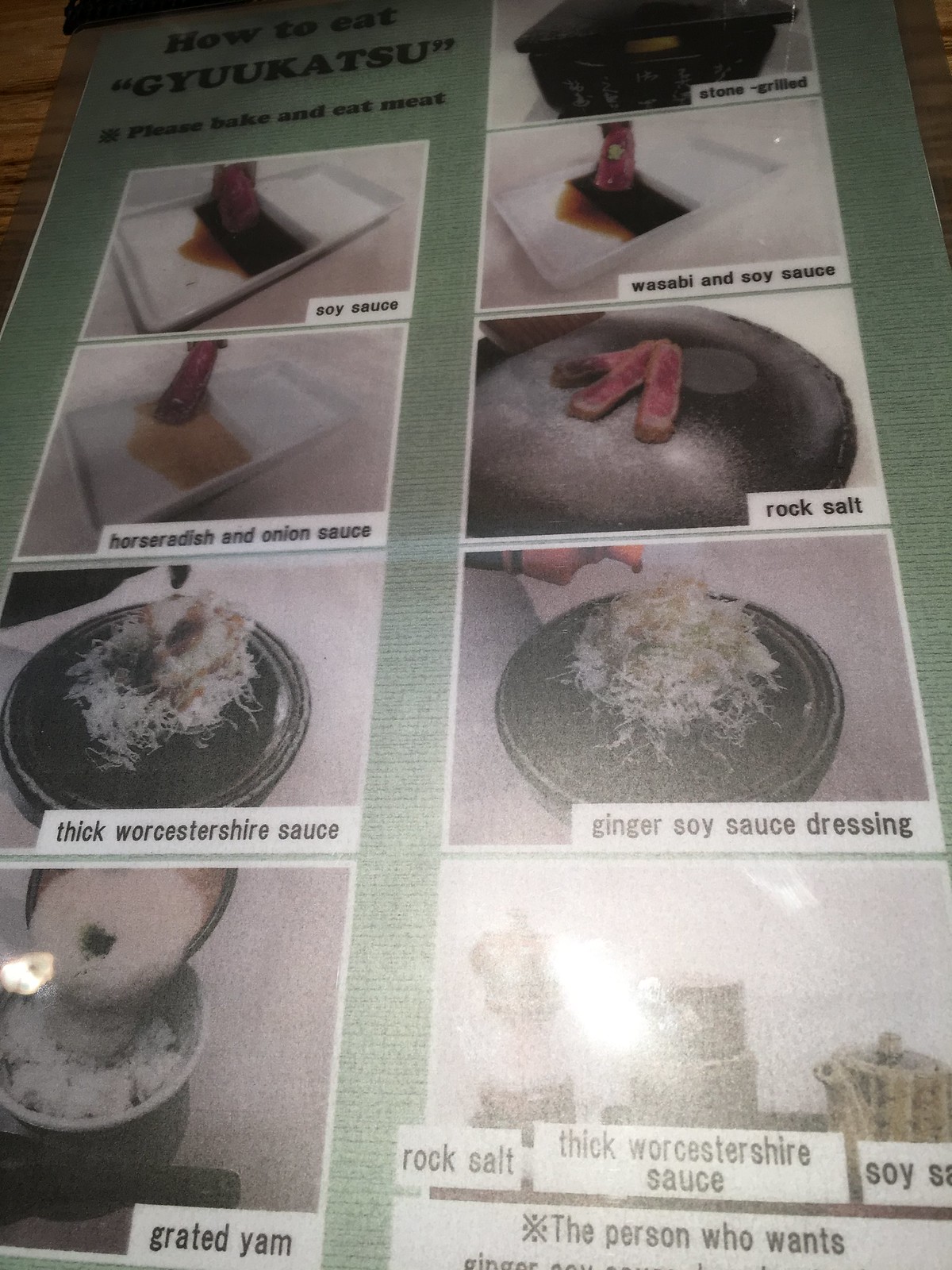This is a photograph of an instructional poster on how to eat "Gyukatsu," a Japanese dish. The poster has a green background and features detailed instructions along with images of various condiments and accompaniments. 

At the top left, in black letters, it reads, "How to Eat 'GYUKATSU'." Directly below this title, it instructs, "Please Bake and Eat Meat."

The poster is divided into two columns, each containing a series of photographs with descriptive labels:

**Left Column:**
1. A square plate filled with a dark sauce, labeled "Soy Sauce."
2. Another square plate with a liquid, identified as "Horseradish and Onion Sauce."
3. A round black plate containing a shredded white food, described as "Thick Worcestershire Sauce."
4. A round black bowl with a white rim filled with a substance labeled "Grated Yam." There is a light reflection on this photograph.

**Right Column:**
1. A picture of a black pot, labeled "Stone Grilled."
2. A square white plate with some sauce, tagged "Wasabi and Soy Sauce."
3. A round black plate with meat strips, labeled "Rock Salt."
4. A round black plate with a shredded white substance, labeled "Ginger Soy Sauce Dressing."

At the bottom, there is significant light reflection affecting the visibility of the images. One of the discernible objects is a coffee or teapot with a spout and lid. The tags nearby read "Rock Salt," "Thick Worcestershire Sauce," and a partially cut-off label that appears to be "Soy Sauce."

In black lettering, partially cut off at the bottom, it seems to read, "The person who wants," followed by a word that looks like "ginger," but the rest is obscured.